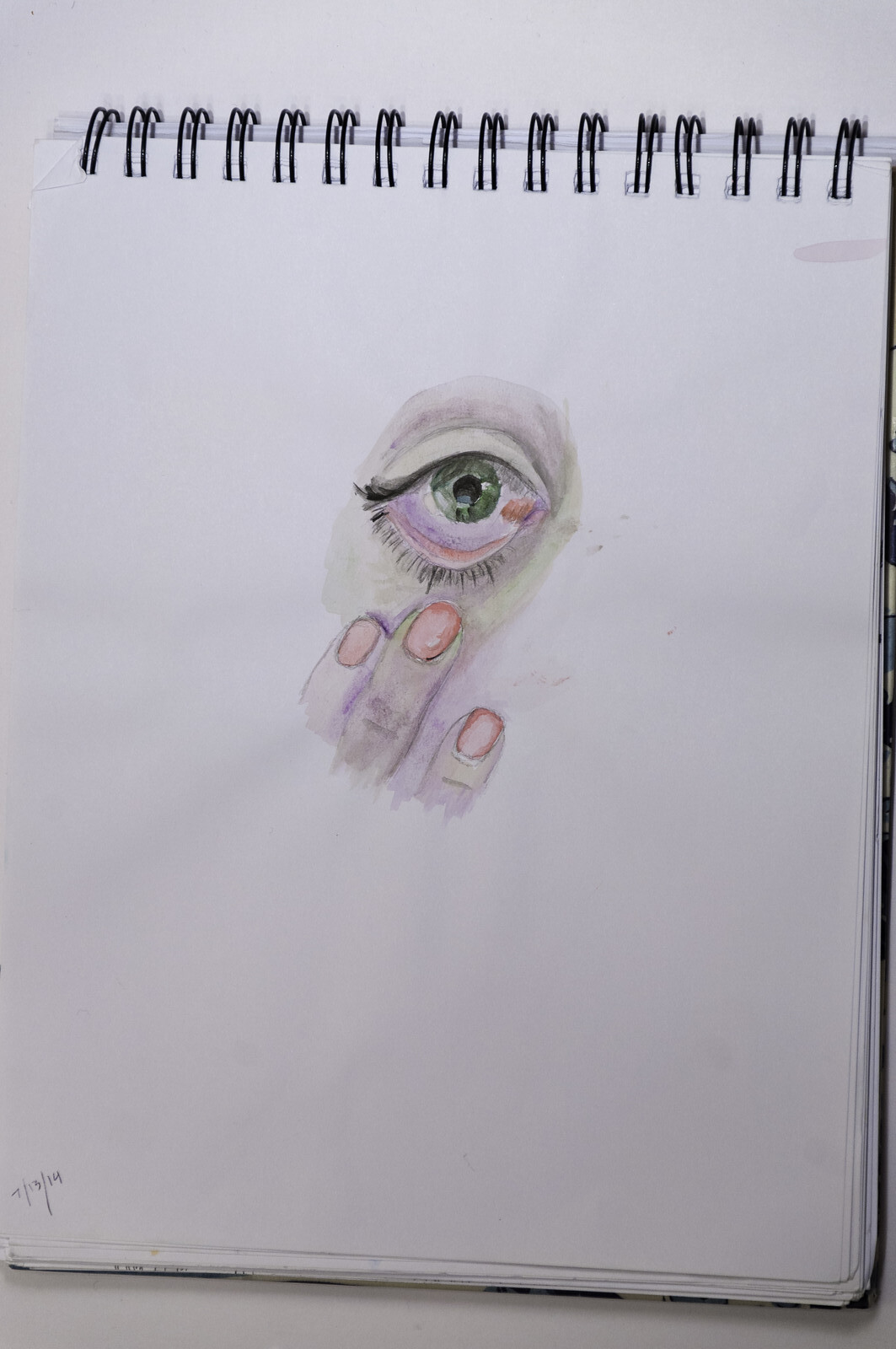This image is a photograph of a detailed drawing, possibly created with colored pencils or watercolors. The artwork features a close-up of a green and white eye, which may be a self-portrait of the artist or simply a depiction of an eye. Surrounding the eye are two hands with a haunting appearance; the fingers, colored in a greenish hue, resemble those of a corpse, while the fingernails are a striking reddish-orange. The eerie, almost otherworldly quality of the composition evokes a sense of mystery and unease.